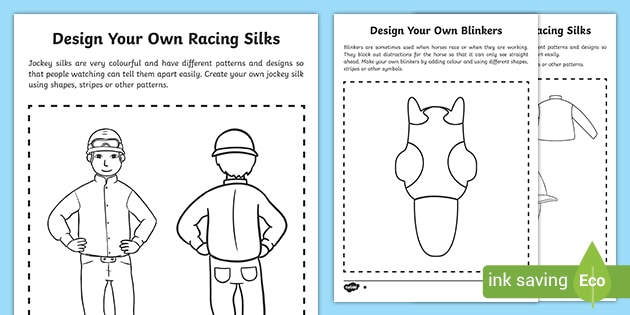The image features a detailed tutorial for designing your own racing silks and blinkers, likely aimed at children. The image is set against a blue backdrop, with three overlapping white sections. The primary section, titled "Design Your Own Racing Silks," showcases an animated jockey from both the front and back, wearing a colorful racing outfit. The jockey, depicted with hands on hips, is surrounded by a dotted line that separates the illustration from accompanying text about the vibrant and patterned nature of jockey silks.

To the right, another section is titled "Design Your Own Blinkers," showing an outline of a horse's head with the blinker headgear, also encased in dotted lines. The third sheet, partially obscured by the blinkers page, features more jockey racing silks, emphasizing the creative and colorful aspect of the activity. The lower right of the image includes a note in a green border that intriguingly states, "ink-saving economy equals a shark."